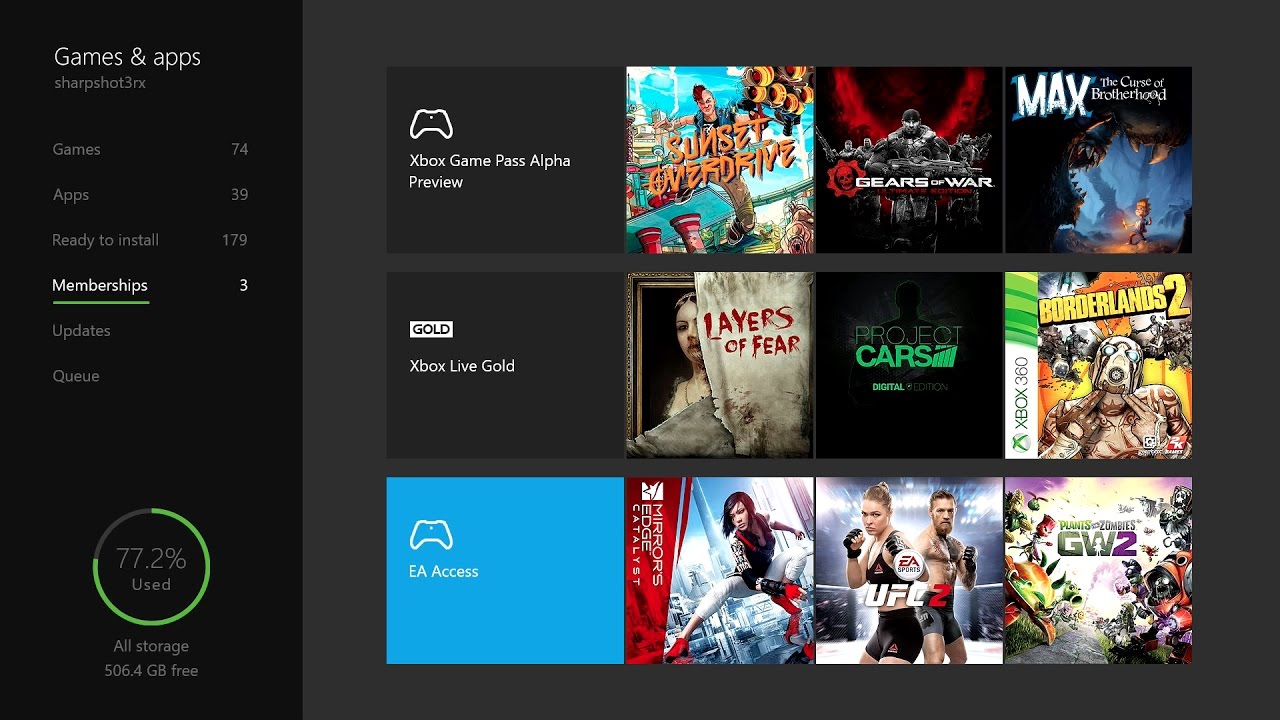The image showcases a detailed screen capture of a video game management interface, likely from an Xbox or Steam platform. Dominating the view is a large, dark gray box. In the top left corner, a black box with white text displays "Games & Apps," followed by “Sharp Shot 3RX.” Below this, it states "Games: 74, Apps: 39," and indicates "179 items ready to install."

Directly underneath, "Memberships" is highlighted with a green underline, listing a total of "3" memberships. Below that, the "Updates" section is mentioned. Further down, a large green circle almost completely filled up shows "77.2% used," near the label "All storage: 506.4 GB free."

To the right, the interface displays various sections such as "Xbox Game Pass Alpha Preview," alongside a list of games including "Sunset Overdrive, Gears of War, and Max: The Curse of Brotherhood." Further down, other memberships are detailed with the respective titles "Xbox Live Gold" and "EA Access," the latter in a distinct blue box, contrasted with the standard medium gray of other memberships.

Under these categories, more games like "Layers of Fear," "Project Cars," "Borderlands 2," "Mirror's Edge: Catalyst," "UFC 2," and "Plants vs. Zombies: GW2" are listed in columns, showcasing a diverse range of titles available or installed.